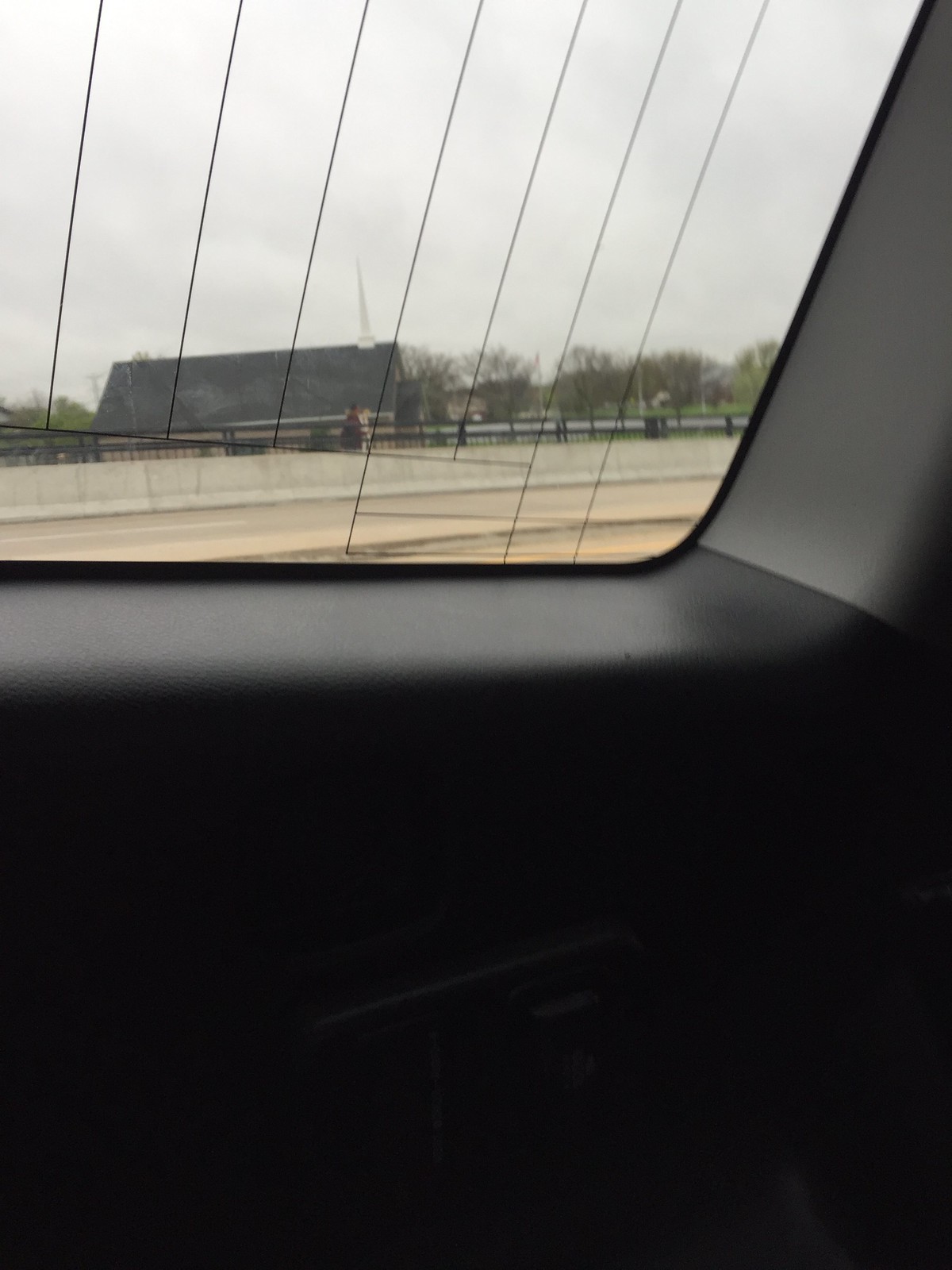In this photograph taken from the interior of a vehicle, the image captures a view out of the car’s window, revealing the gray plastic trim outlining the window itself. Below this, the black plastic of the door panel is visible, but it fades into darkness as the lower part of the car's interior is shrouded in shadows. The window features faint black defroster lines stretching vertically. Outside, a gray paved road and a gray-colored divider are discernible. Across the road, a brown building with a gray roof stands prominently, adorned with a white steeple that pierces the cloudy sky above. In the background, a barren tree line adds a stark contrast to the overcast atmosphere.